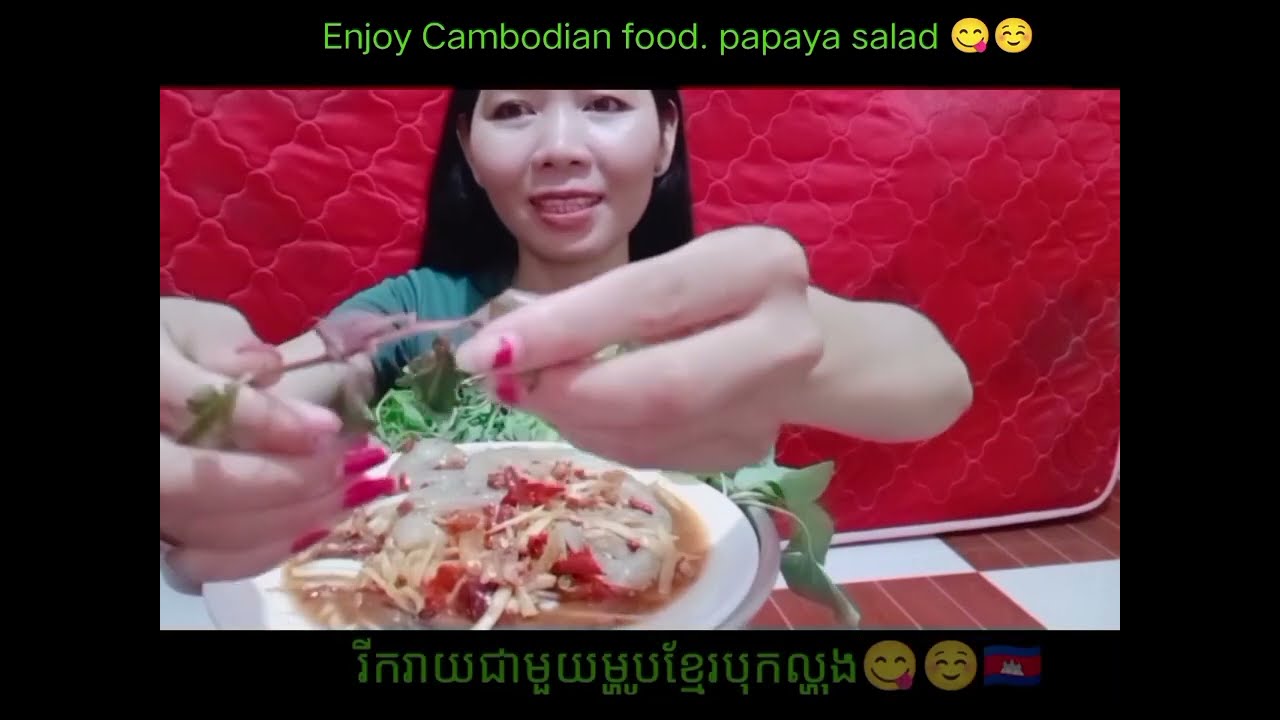The image showcases a light-skinned Asian woman with long black hair and pink fingernails, wearing a green shirt. She is centrally positioned, holding a leafy vegetable in one hand. In front of her, there is a white plate or bowl containing what appears to be Italian food with red and green ingredients, possibly tomatoes and green leaves. The surrounding setting includes a floor with white and brown tiles and a red fabric backdrop featuring a wavy diamond pattern that covers the wall. This scene is framed by a thick black border adorned with emojis. At the top, green text reads "Enjoy Cambodian food, papaya salad," accompanied by two yellow emojis—one with its tongue sticking out and the other blushing. At the bottom, there is text in a language that appears to be Korean, accompanied by more emojis and a flag, possibly indicating the country related to the language.